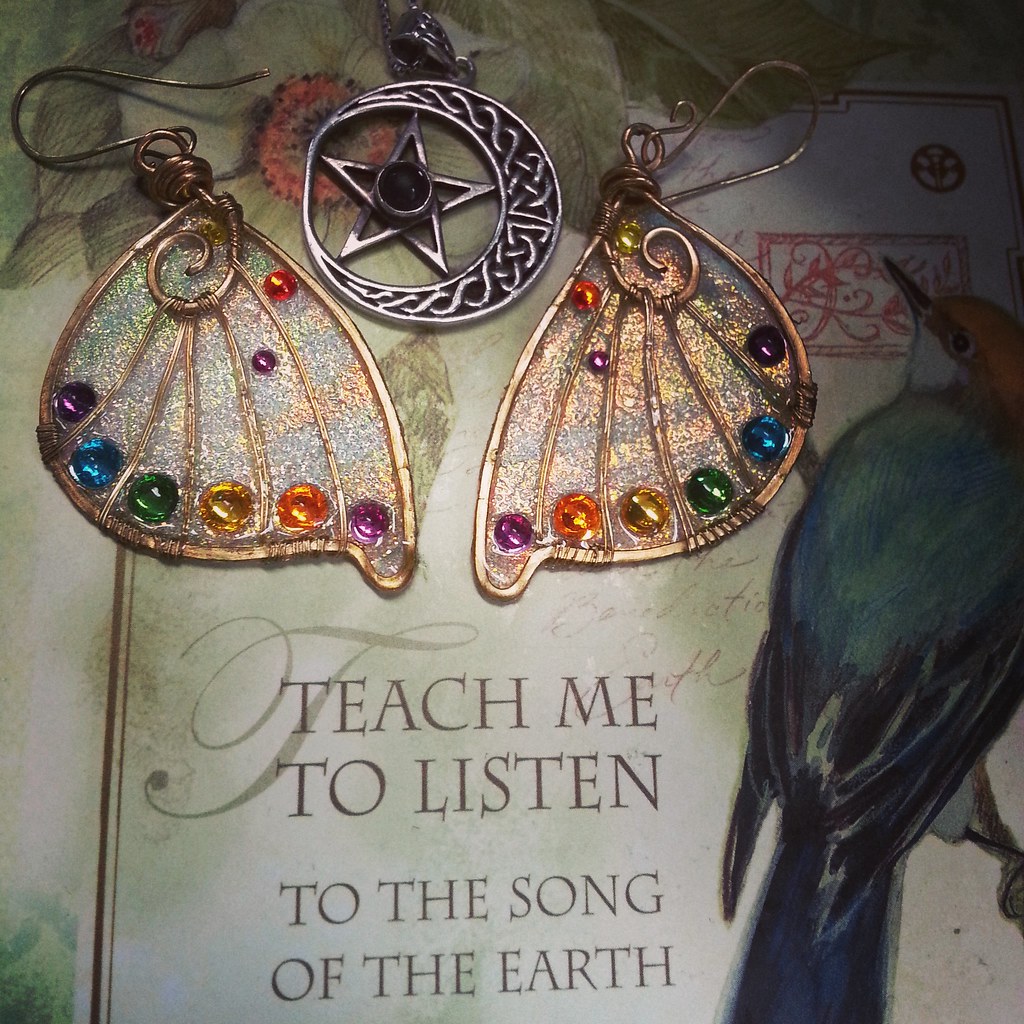The image depicts a display likely from a store or exhibition of handmade jewelry, with a trio of ornate earrings set against a painterly backdrop. At the forefront, a central silver earring features an intricate design of a crescent moon with a star nestled inside. Flanking this centerpiece are two gold earrings that resemble butterfly wings, adorned with a multitude of colorful gemstones. Beneath these stunning pieces, the background features a softly blended white and green surface with a hand-painted green bird with a yellow head positioned towards the bottom right, visible from behind with its head turned upwards. Overlaying this backdrop, the inscription in purple reads, “Teach me to listen to the song of the earth.” This single, poetic sentence combines with the artistic and whimsical elements of the earrings and the painted bird to create a visually arresting and cohesive display.